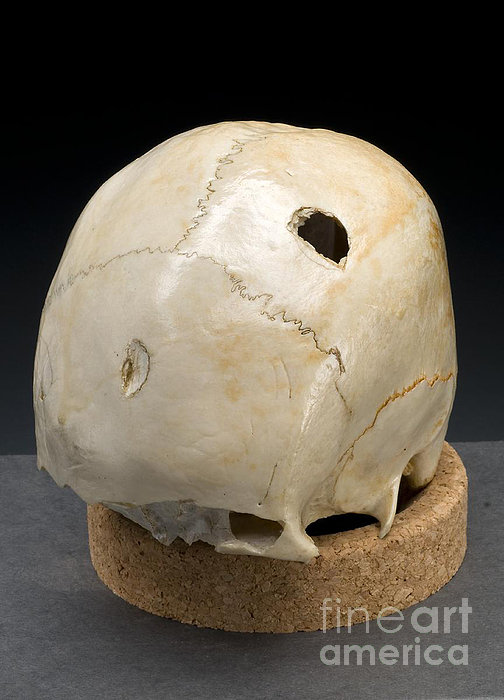This vertically aligned rectangular image captures an artistic or historical artifact: a white, slightly beige animal skull featuring jagged cracks and an eye cutout that reveals a solid black background. The skull exhibits a smooth, almost polished surface that reflects the camera light, highlighting its intricate details. It rests on a brown, wood-stained circular pedestal placed on a matte gray tabletop. The scene is set against a stark black backdrop, giving the skull a dramatic and intense look. In the bottom right corner, the light gray text reads "Fine Art America," indicating the artwork's marketplace or print origin.